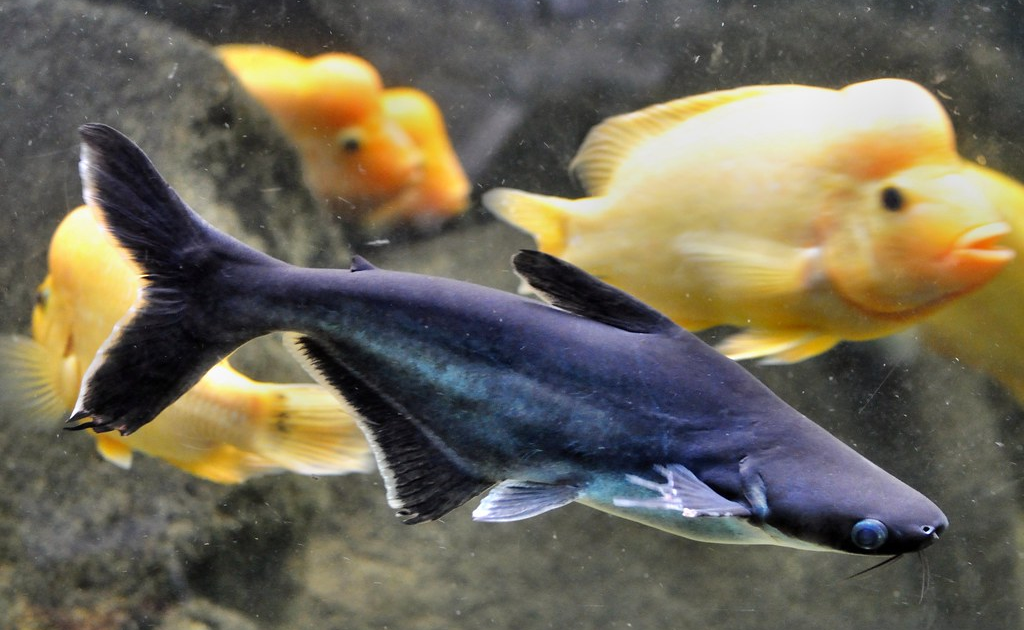This photograph captures a vibrant underwater scene within a fish tank or aquarium, showcasing a variety of colourful fish against a backdrop of gray rocks. Central to the image is a small blue catfish, easily identifiable by its whiskers, bulging blue eyes, and a lighter belly with black, white-tipped fins. This catfish is prominently positioned in the foreground, making it the main focal point.

Surrounding the catfish are four to five yellow-gold fish, resembling goldfish, with distinctive black, beady eyes and a notable bulbous structure on their foreheads, reminiscent of a knot or a quirky hairdo. These goldfish exhibit a striking colour likened to that of a baby duck. The tank's setting includes some visible gray rocks, particles floating in the water, and a generally muted background, highlighting the vivid colours and details of the fish.